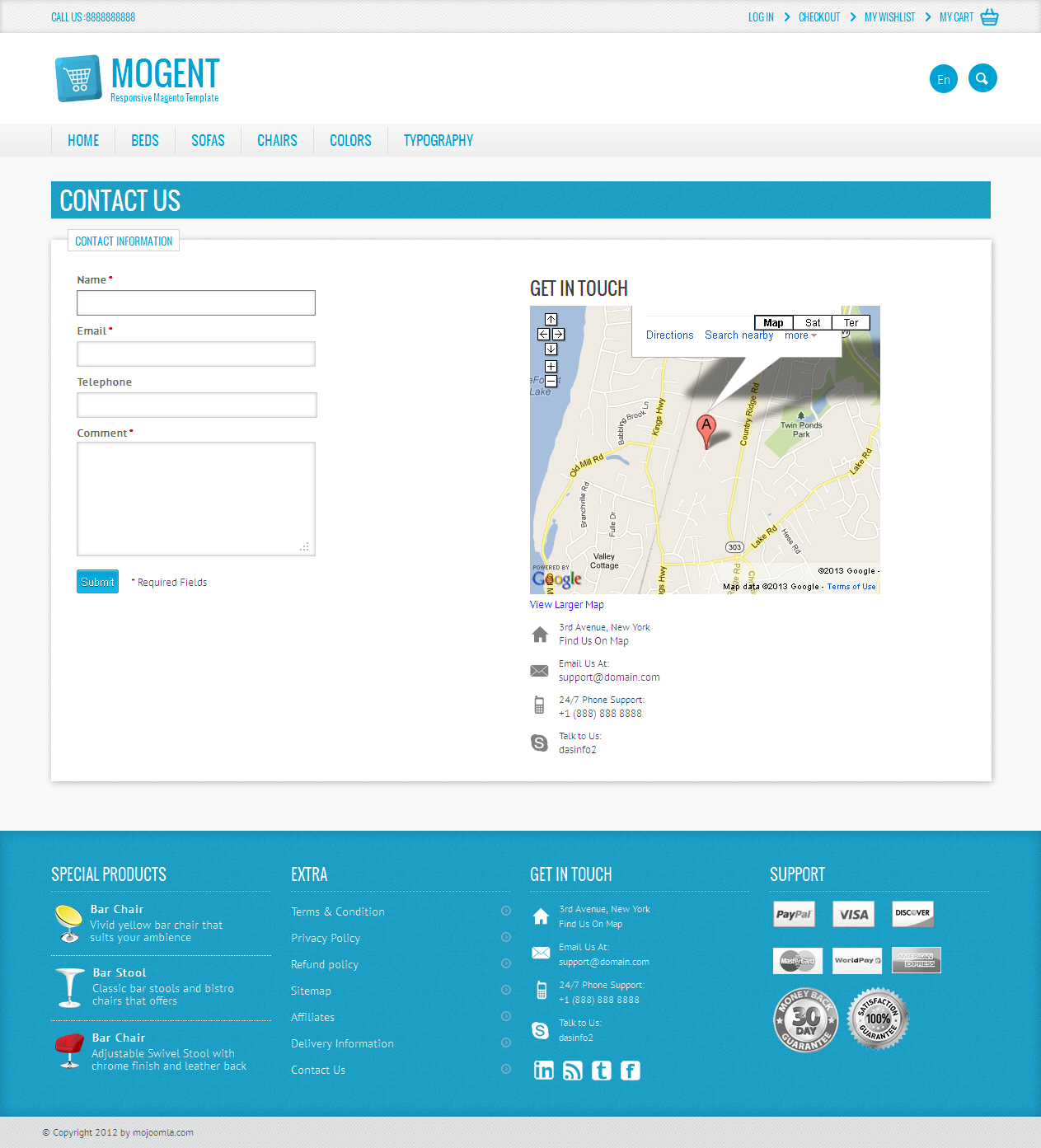This is a detailed screenshot from the Mogent website. At the very top, there's a navigation bar with blue text options including "Call," "Log In," "Check Out," "My Wish List," and "My Cart." Adjacent to this text, towards the left, the brand name "Mogent" is displayed next to a grocery cart logo. To the right of the logo, there are two circular icons: one labeled "EN" presumably for language selection, and the other featuring a magnifying glass, indicating a search function.

Below this top bar, there's a white navigation menu listing various categories such as Home, Beds, Sofas, Chairs, Colors, and Typography. Directly beneath this menu, on a blue bar with white text, there is a "Contact Us" section. 

The contact area consists of several text boxes for visitors to input their name, email, telephone, and comments, followed by a submit button. Next to this form, there's an embedded map with "Get in Touch" written in black text. Below the contact section, additional sections provide various types of information.

At the very bottom of the page, another blue box contains links to "Special Products" like "Bar Chair" and "Bar Stool," along with icons representing different types of chairs. This area also includes sections for "Get in Touch" and "Support."